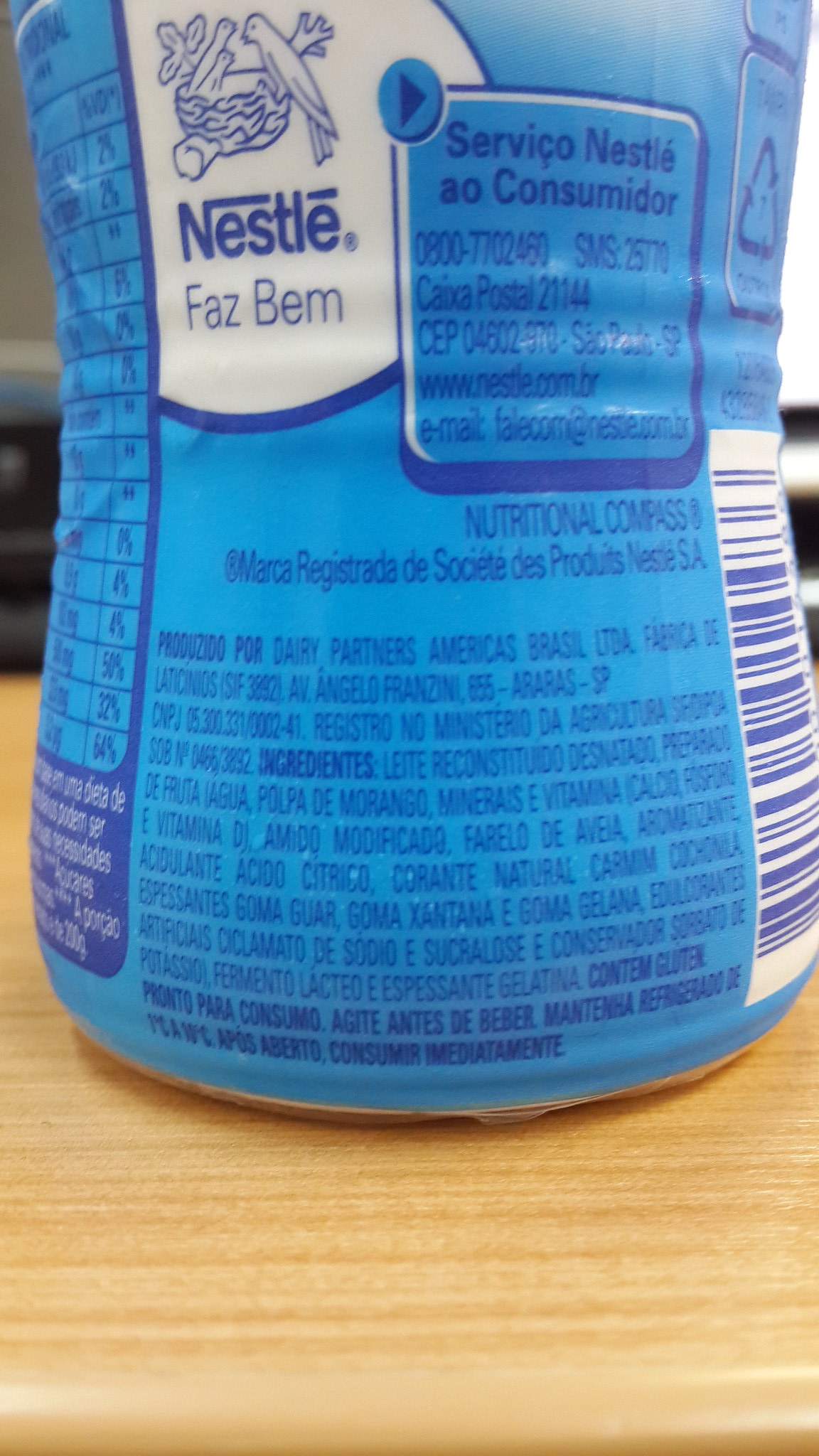This photograph shows a blue plastic bottle sitting on a light tan wood-grained surface. The bottle is adorned with detailed Nestle branding. At the top left of the label is the Nestle logo featuring a blue bird and nest on a white background. Below, in dark blue letters, the text reads "Nestle FASBEM." The label includes a prominent white semicircle displaying a dark blue Nestle logo. Adjacent to this is a blue square containing consumer information, including a postal code and mention of Sao Paulo, SP. The bottle is likely a dairy product, evidenced by the presence of further nutritional information and produced by Dairy Partners Americas Brazil, Limitada. Surrounding this text are additional data and ingredient lists, all printed in dark blue. The photograph also captures parts of a wooden table and a faint, neutral background, adding context to the setting.